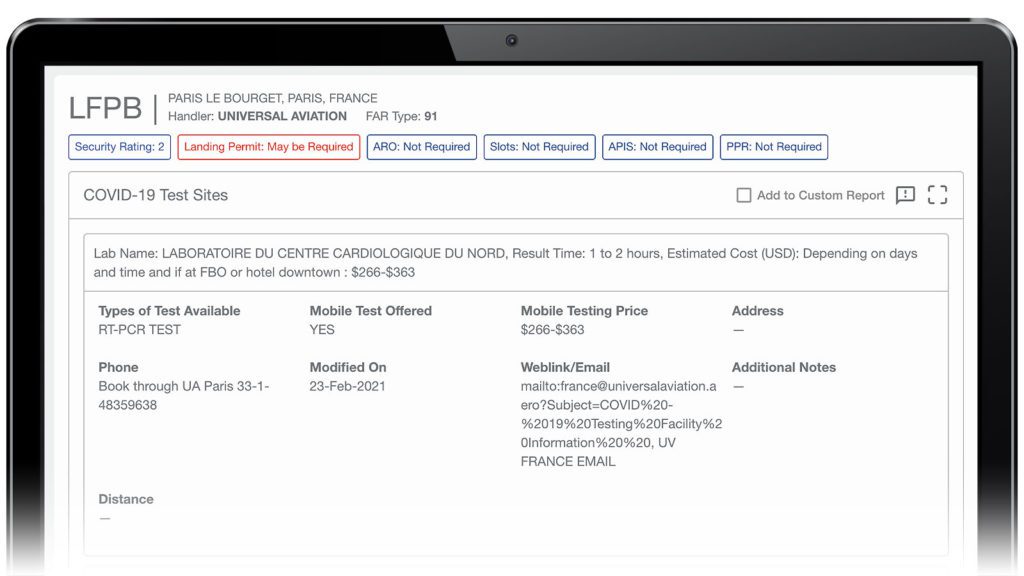In this image, the screen displays logistical information for LFPB (Paris Le Bourget Airport) located in Paris, France. It mentions the handler, Universal Aviation, and provides flight-related details including the F.A. Aerotype 91 code and a security rating of 2. Additional notes indicate that a landing permit may be required, while arrow slots and APIS are not necessary. The text also mentions "Carbonizing Test Sites" with the lab name "Lucentac Cardiologic" and personnel named Bernard. Test results can be expected within 1-2 hours, and the estimated cost varies depending on the day and time. If conducted at an FBO (Fixed Base Operator) or downtown hotel, the price ranges from $266 to $363. Types of tests available include the Aerotypic PCR Test and Mobile Test of Agiles, with mobile testing priced at $266.